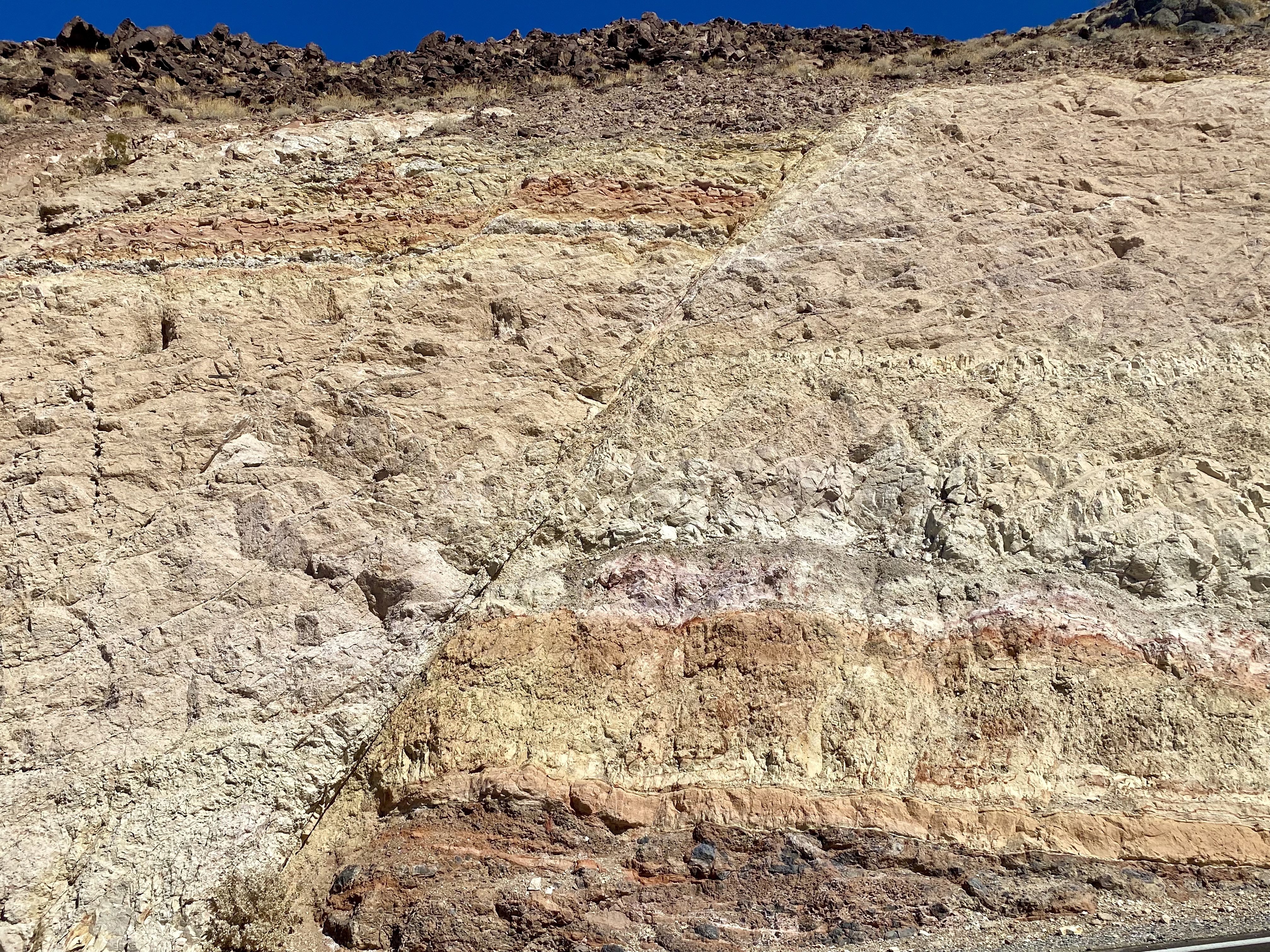The image depicts a rugged cliff-like rock formation with a variety of discolored rocks that suggest past water presence. Predominantly composed of sandy and earthy hues, the rocks exhibit a rich stratification of colors, ranging from dark brown and beige to light tan and nearly white. This picturesque yet arid landscape, captured from a lower perspective looking upwards, features a deep blue sky noticeable just at the top edge of the frame, hinting at the height of the formation. The scene is devoid of any people or animals, emphasizing its desolate, desert-like quality. The rocky surface appears rough and unscalable, accentuated by patches of dirt and dryness, while a touch of green vegetation is discernible only at the very top, probably near the land's surface. These stacked rock layers or excavation lines create a compelling visual of natural geology, suggestive of sedimentary processes over time.